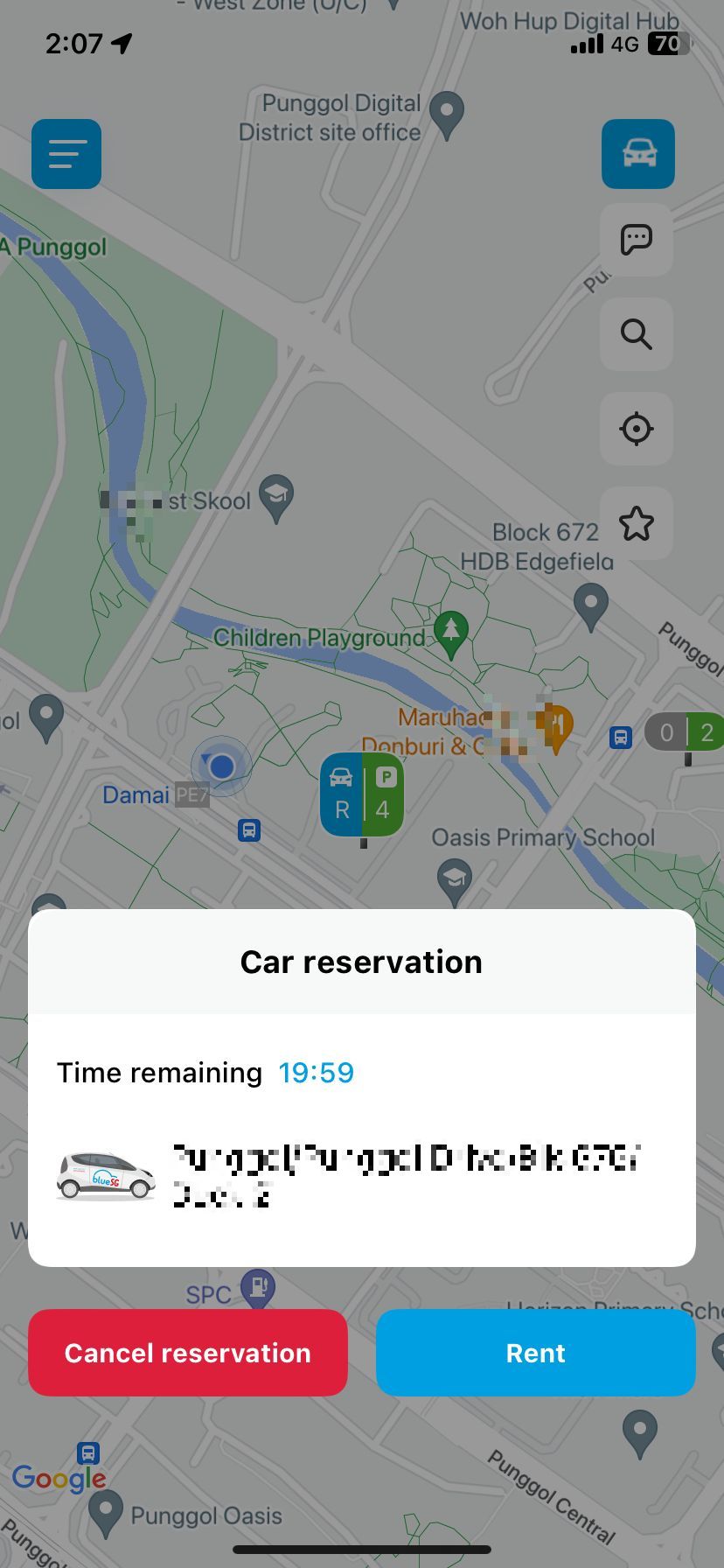The image depicts a smartphone screen displaying a car reservation app with an open map in the background. Overlaying the map, there is a white pop-up box at the bottom of the screen that shows the message "Car Reservation Time Remaining: 1959." The numeric "1959" is highlighted in blue, while the rest of the text is in black. There is a small image of a car within the pop-up box, with car details obscured in mosaic to protect personal information.

Below the text, there are two action buttons: one red button labeled "Cancel Reservation" situated on the bottom-left corner, and one blue button on the bottom-right corner whose label is not fully visible in the description but could be for confirming the reservation.

The map in the background contains several colorful icons and certain parts of the map are covered in mosaic to conceal specific locations. On the top-left corner of the app, there is a main menu icon featuring three horizontal white lines on a blue background. On the top-right corner, there is a blue car icon with a white outline. Below this icon, there are additional buttons: a message icon, a search icon, a current location icon, and an "Add to Favorite" icon, all drawn in black on a white background.

Overall, the image captures a functional and interactive car reservation app interface with multiple navigation and action buttons designed for user convenience.